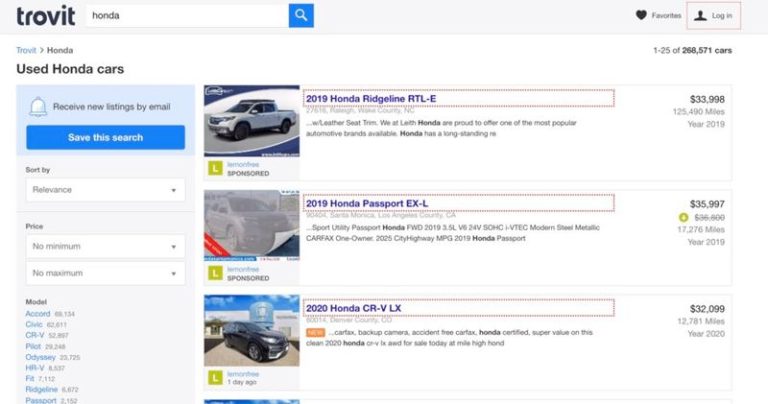A detailed caption for the image described:

"The webpage displayed is from Trovit, a site dedicated to listing used cars for sale. The top left corner features the Trovit logo next to a search bar where 'Honda' is entered. To the right of the search bar, there are options for 'Favorites' and 'Log In'. 

Below this header, the left sidebar repeats the search details: 'Trovit', 'Honda', 'used Honda cars'. There is also an option to receive new listings by email, indicated by a bell icon, and a button to save the current search. Listings are currently sorted by relevance, which can be changed via a drop-down menu. Filters for price range (with no minimum and maximum values selected) and model type are available. Under the model filter, several Honda models are mentioned: Accord, Civic, CR-V, Odyssey, Fit, Ridgeline, and Passport, though some details are blurry.

In the main section of the page, three vehicles are prominently featured, each with an accompanying photo on the left. The first listing is for a '2019 Honda Ridgeline RTL-E' featuring leather seat trim and described as a highly popular automotive brand. The second listing is also a Honda vehicle from 2019, though further details are not visible in the description."